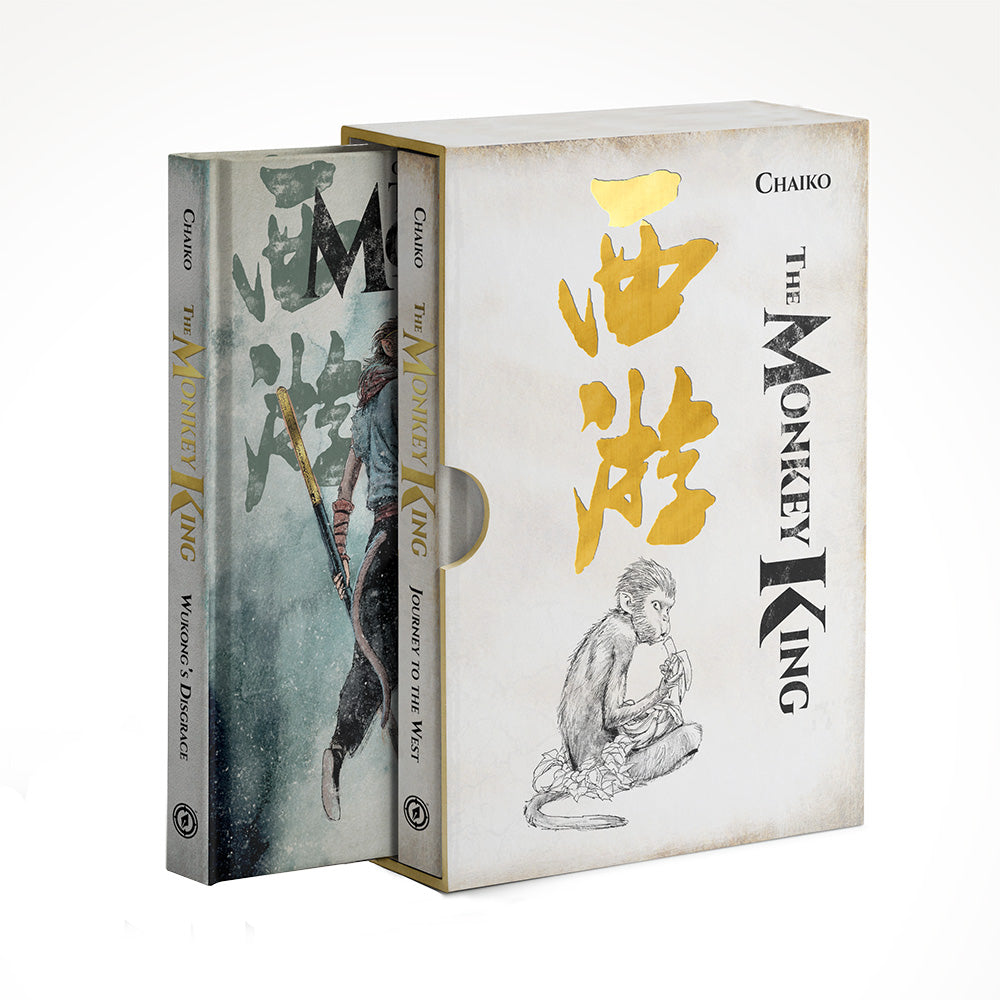This high-resolution, professionally-taken photograph displays a square-shaped box set against a very light beige background, which might be in an art studio or edited out. The set contains two books housed in a worn-looking, beige-gray cardboard sleeve. The front of the sleeve prominently features an illustration of a monkey in black ink, eating a banana and looking over its right shoulder. Next to the monkey, black text reads "The Monkey King," with additional Chinese text written in gold lettering also visible.

The two books inside the sleeve are titled "Journey to the West" and "Wu Kong's Disgrace," each having "The Monkey King" written in black text on their spines. The back book, "Journey to the West," is partially slid out, showcasing its spine clearly. The detailed design and text emphasize the artistic and literary significance of the set.